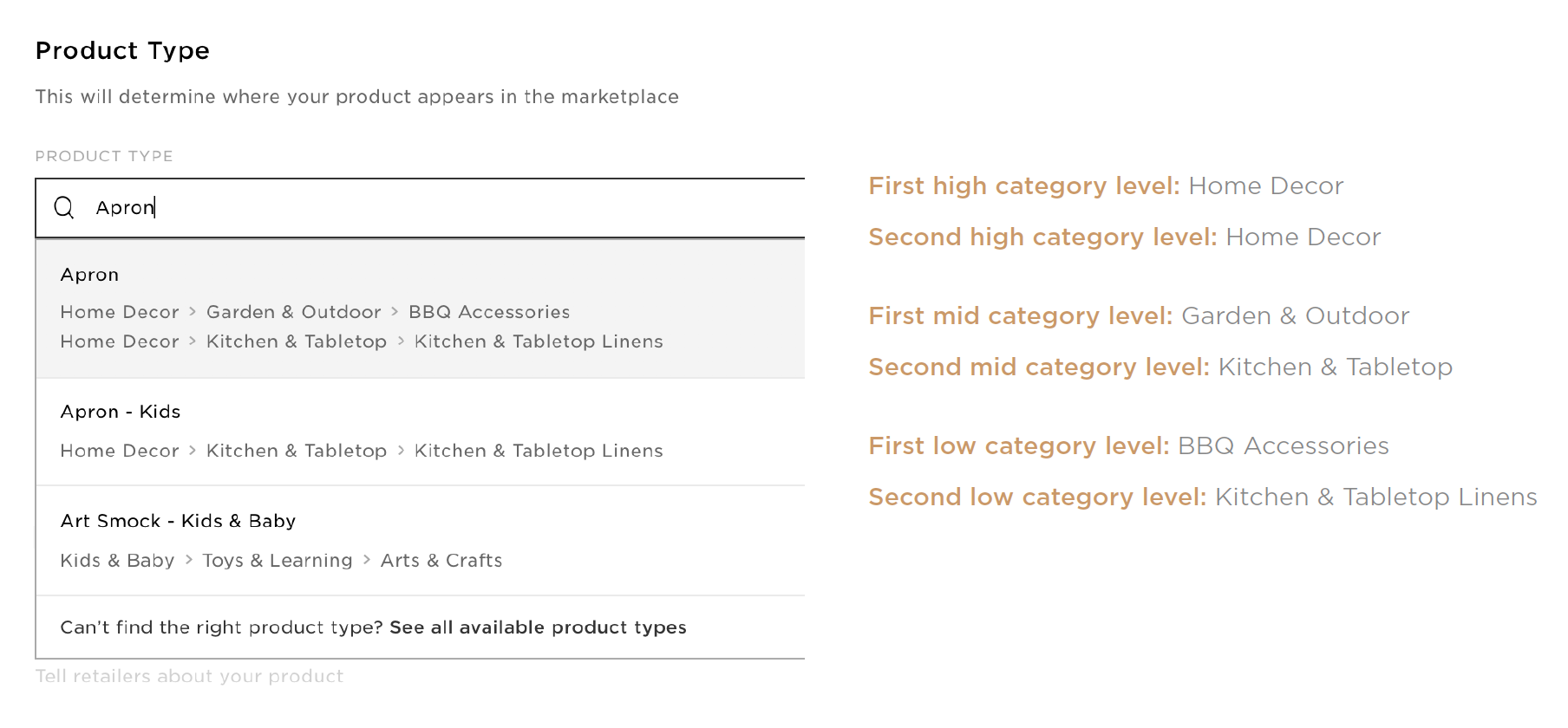The image is a detailed screenshot of a digital marketplace interface specifically for categorizing products. In the top left corner, the text "Product Type" appears. Directly below, there's a note stating, "This will determine where your product appears in the marketplace." Beneath this is another label, "Product Type," accompanied by a search box where the user is currently typing "apron."

As the user types "apron," a dropdown menu expands with several categorized options:

1. **Apron**:
    - **Home Decor**
        - Kitchen & Tabletop
            - Kitchen & Tabletop Linens
    - **Gardening & Outdoor**
        - Barbecue Accessories

2. **Apron for Kids**:
    - **Home Decor**
        - Kitchen & Tabletop
            - Kitchen & Tabletop Linens

3. **Art Smock for Kids & Baby**:
    - **Kids & Baby**
        - Toys & Learning
            - Arts & Crafts

At the bottom of the dropdown, the text reads, "Can't find the right product type? See all available product types." To the right of the screen, text in a goldish font says, "First High Category Level: Home Decor." Below that, in gray font, it reads, "Second High Category Level: Home Decor." 

Further down, it states:

1. **First Mid-Level Category Level**: Gardening & Outdoor (in gray font)
    - **Barbecue Accessories** (First Low Category Level)

2. **Second Mid-Level Category Level**: Kitchen & Tabletop (in gray font)
    - **Kitchen & Tabletop Linens** (Second Low Category Level)

This comprehensive categorization system is designed to guide users in effectively organizing their products for optimal marketplace visibility.